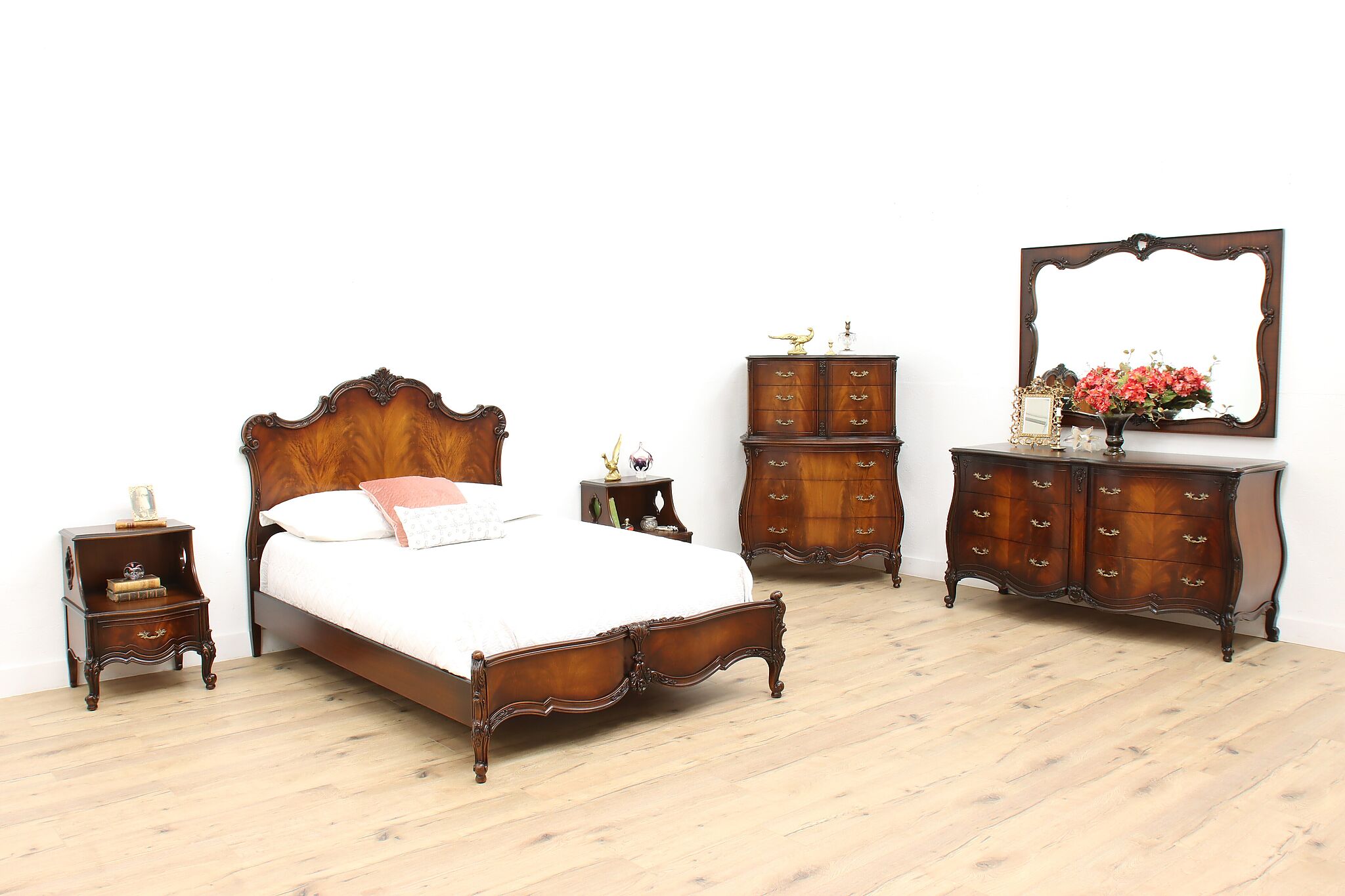This image features a pristine bedroom set against stark white walls with a light oak or birch-colored floor, exhibiting minor knots. The focal point is a magnificent deep mahogany double bed with an elaborate, pointed headboard, draped in a crisp white linen bedspread. A notable peach or pink pillow is placed centrally among two larger white pillows and a smaller pillow in front. 

On each side of the bed are two identical, ornate antique bedside tables. These beautifully crafted tables feature curved legs and brass or gold handles, with one drawer and an open shelf below. One nightstand holds indistinguishable items while the other displays several books and a glass.

In the far left corner stands a stately woman’s dresser with three large drawers beneath and two upper doors. Atop this elegant piece rest two types of glassware items. Adjacent to this, in the far right corner, is a matching lower dresser with similar brass handles. This dresser supports a framed picture and a vase filled with pink or orange flowers, complemented by a large, ornately framed mirror that spans the width of the dresser and shares the same deep mahogany tones. The cohesive aesthetic and intricate details underscore the room's antique elegance.